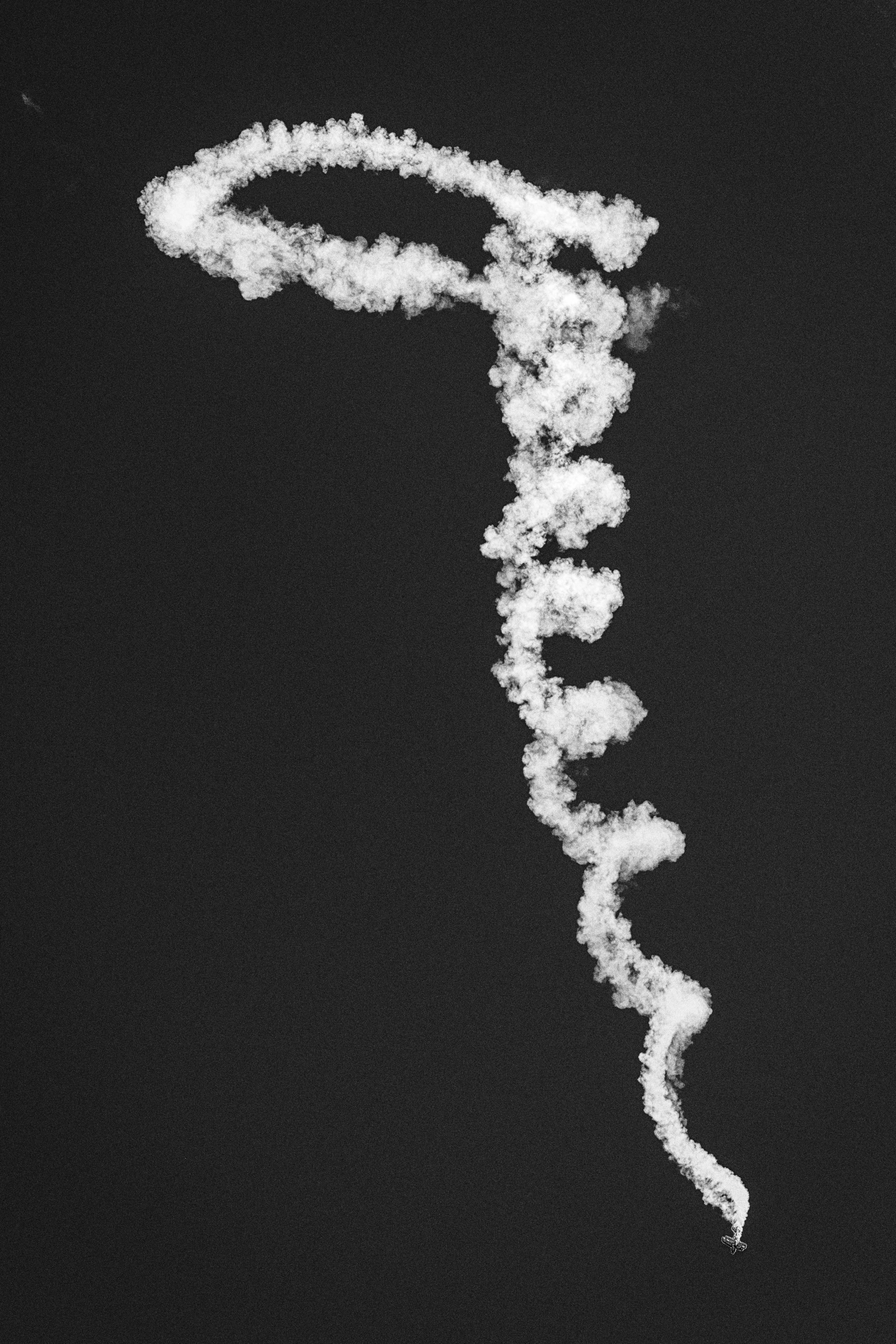The image presents a stark black background featuring a prominent trail of smoke or vapor. Originating from a small, nearly indiscernible source possibly resembling a plane or vehicle at the bottom right, the smoke extends upwards along the right side of the picture. As it ascends, the smoke, which is primarily white with subtle light gray tinges around its edges, swirls in a manner reminiscent of an old telephone cord or a pig's tail. The swirling motion creates an intricate pattern, including a significant loop at the top, giving it the appearance of a chemtrail or an artistic rendition of either smoke or a fuzzy material. The curling formation continues upwards, creating a sense of movement and dynamic flow that contrasts sharply with the pitch-black background. The focus remains on the elongated, spiraling trail which features roughly eight discernible swirls before culminating in a distinct loop, emphasizing the complex, swirling nature of the white and gray interplay against the void-like backdrop.